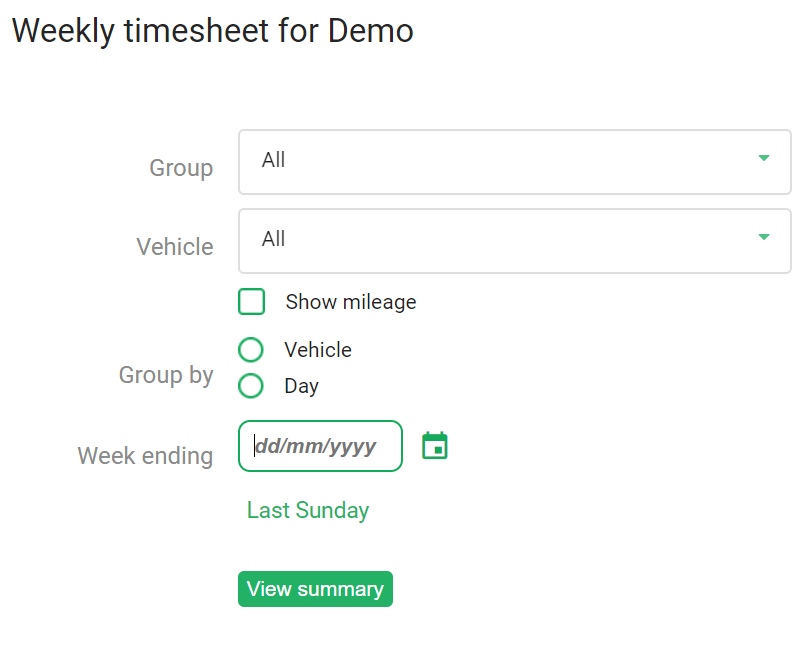The image displays a detailed weekly timesheet interface designed for demonstration purposes. At the very top, the bold, capitalized text reads "WEEKLY TIMESHEET FOR DEMO." Below this heading, there are a series of dropdown menus and checkboxes:

- **Group**: Dropdown menu set to "All" with a green tab indicating that it is adjustable.
- **Vehicle**: Another dropdown menu, also set to "All" with a green tab.

Further along the interface:

- A **green square labeled "Show Mileage"** box allows users to toggle mileage tracking.
- The text **"Vehicle"** again appears, next to a circular icon with a green border and a clear center indicating an option selection.
- **Group By**: Followed by a circle that likely functions as a selectable filter.
- **Day**: Another selectable option for organizing the timesheet data.
- Under **Week Ending**, a format "DD/MM/YYYY" is indicated in a green rectangular box, with an adjacent clickable calendar icon to select the date.
- Below the calendar, there is the label "Last Sunday" in green.

Finally, at the bottom right, a green rectangular button with white lettering prominently displays "VIEW SUMMARY," allowing the user to generate a summarized view of the entered timesheet data. The entire layout is presented against a clean, white background.